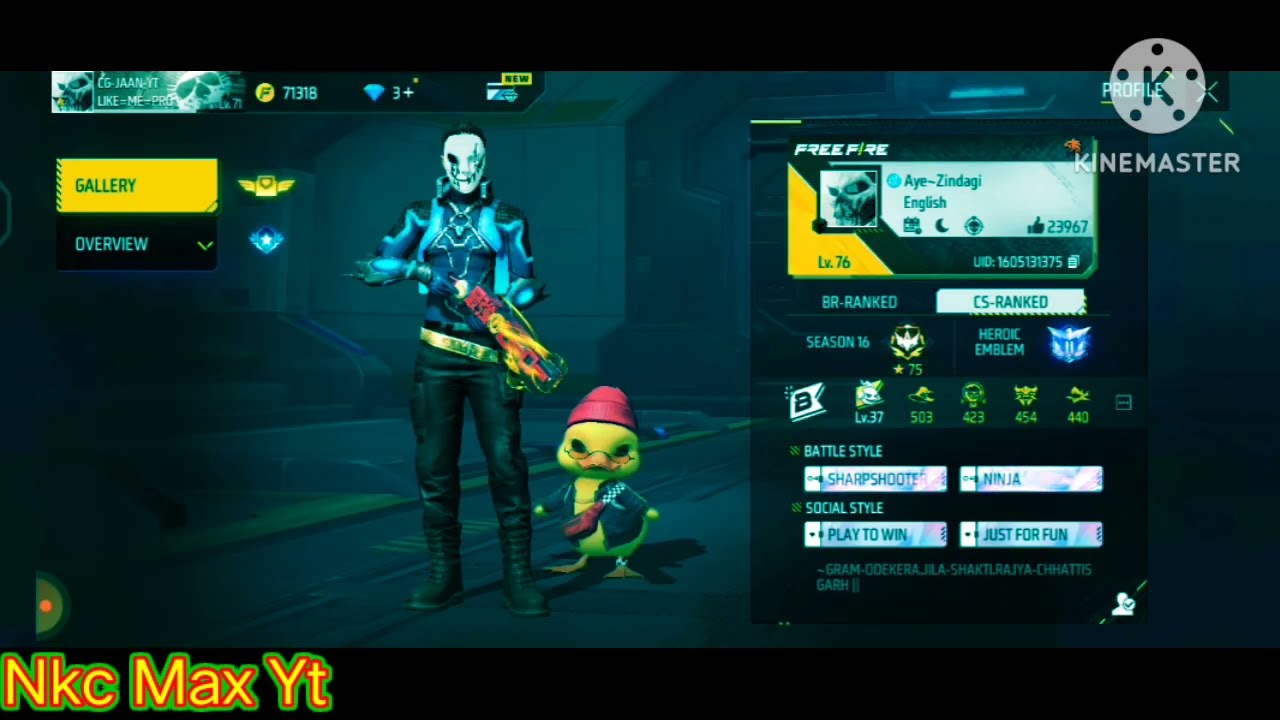This full-color digital image is a screenshot from a video game. The screen has black borders on the top and bottom, with the lower left-hand corner displaying "NKC max YT" in yellow letters with a green outline. The upper right-hand corner features a watermark for KineMaster: a white circle with five white paper hole punches and a large letter "K" cut out in the middle. Below this watermark is a rectangular platform displaying player statistics, including a "sharpshooter" battle style and a "play to win" social style.

At the center of the image are two distinct characters. On the left, we see a humanoid figure wearing black boots, black pants, and a leather jacket with light blue squiggly designs on the shoulders and a navy blue section on the stomach area. This character dons a white mask with an evil-looking smile, a red eye with black drips, and a black line through the right eye. They are holding a large gun, which is red with yellow wrapping around the front. To the right of this character stands a small yellow duck wearing a black leather jacket, a red beanie, and glasses on its orange beak. The duck also has something strapped across its chest. The overall scene is dynamic and filled with intricate details that highlight both the characters and the player's in-game statistics.